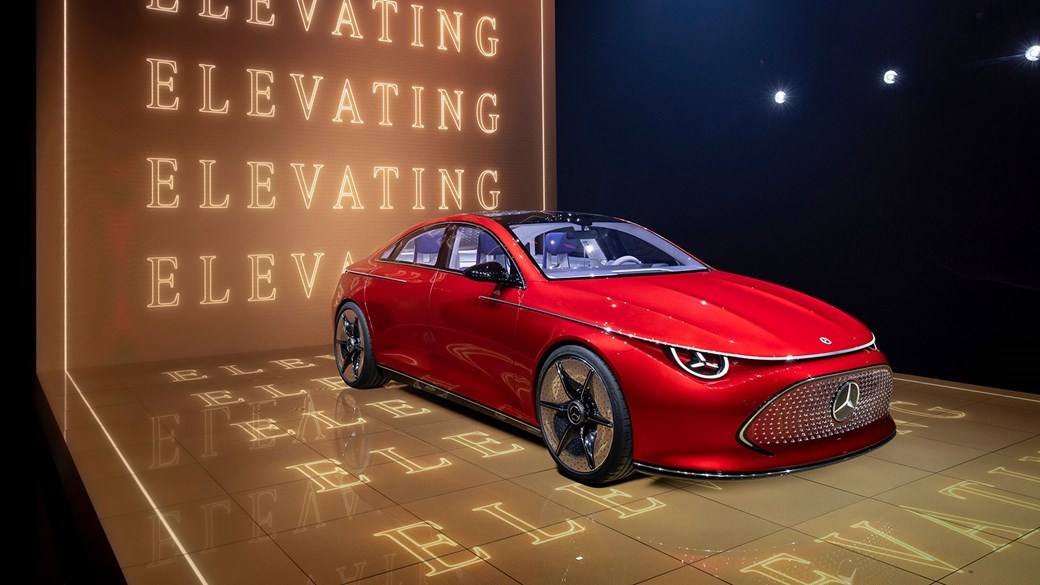The photograph showcases a striking, futuristic red Mercedes-Benz sports car on display. The car features shiny, spiked black rims and a silver grille with a circular emblem at its center. Its interior, visible through large windows, is illuminated with a cool gray-blue tint, highlighting the gray seats. The car is set against a dramatic, dark brass background that transitions from brown to blue near three evenly spaced lights to the right. The stage beneath the car is highly reflective, adding to the spectacle. The background and stage are adorned with repeated, lit-up "elevating" text in a gold-brown neon color, creating an immersive, high-tech atmosphere. This display, devoid of any people, appears to be a high-end showcase, emphasizing the car's luxurious and advanced features.